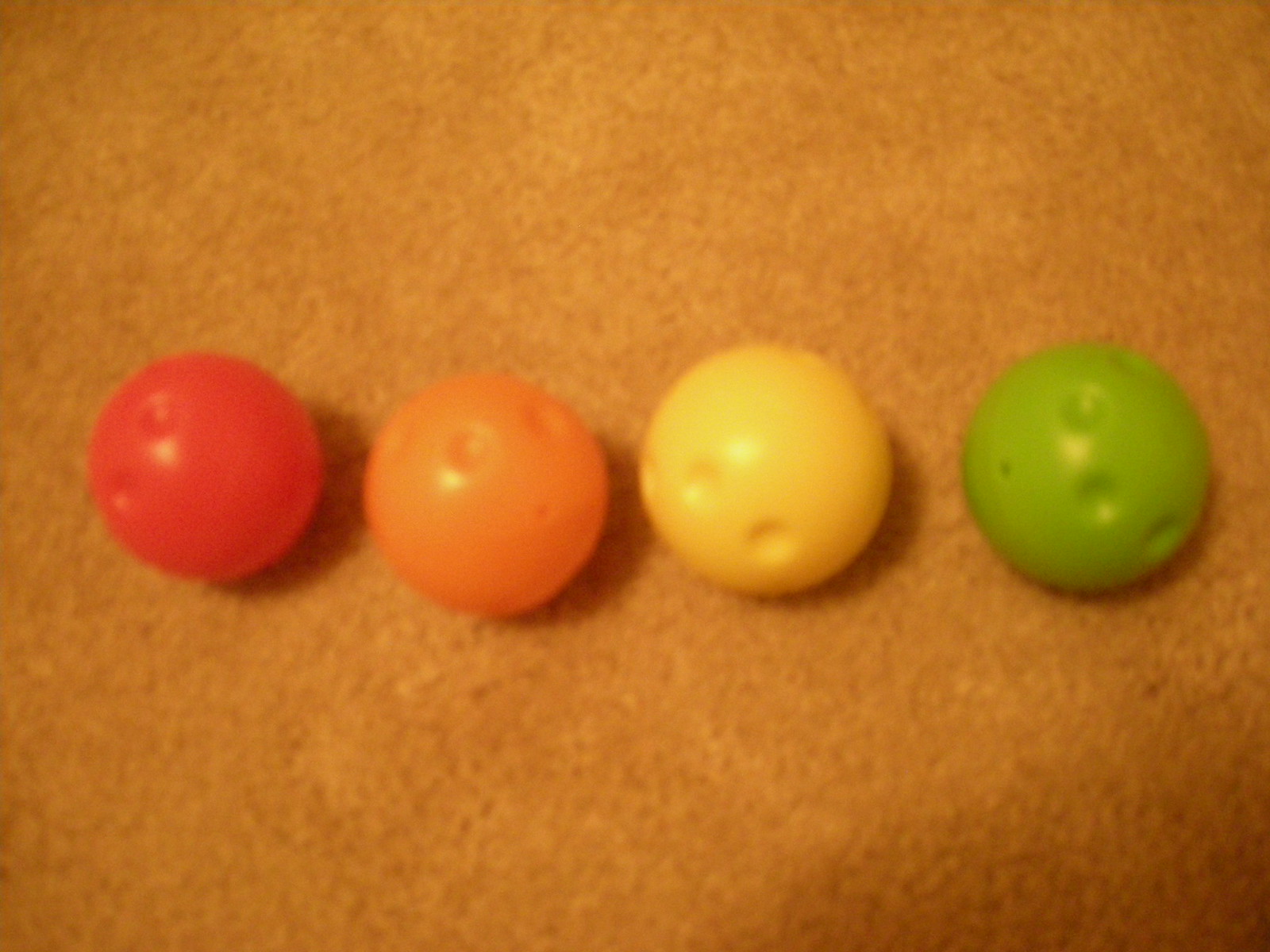This image captures a close-up view of four spherical objects aligned horizontally across the center of a rust-brown and orange background, which appears darker towards the corners with significant shading in the bottom right. The spheres, resembling tactilely soft plastic balls or perhaps wiffle balls due to their dimpled surfaces, are each of a different color: from left to right, red, orange, yellow, and green. Despite the overall poor quality and slight blurriness of the photo, the dimples on each sphere are distinctly visible, suggesting possible indentations for gripping. These indentations are scattered unevenly across each ball, with the red, orange, and yellow balls showing two to three dimples each, while the green ball displays about four. The background surface has an aged, dingy appearance, further accentuated by the shadows and the layout of the spheres, which are not perfectly spaced or aligned.